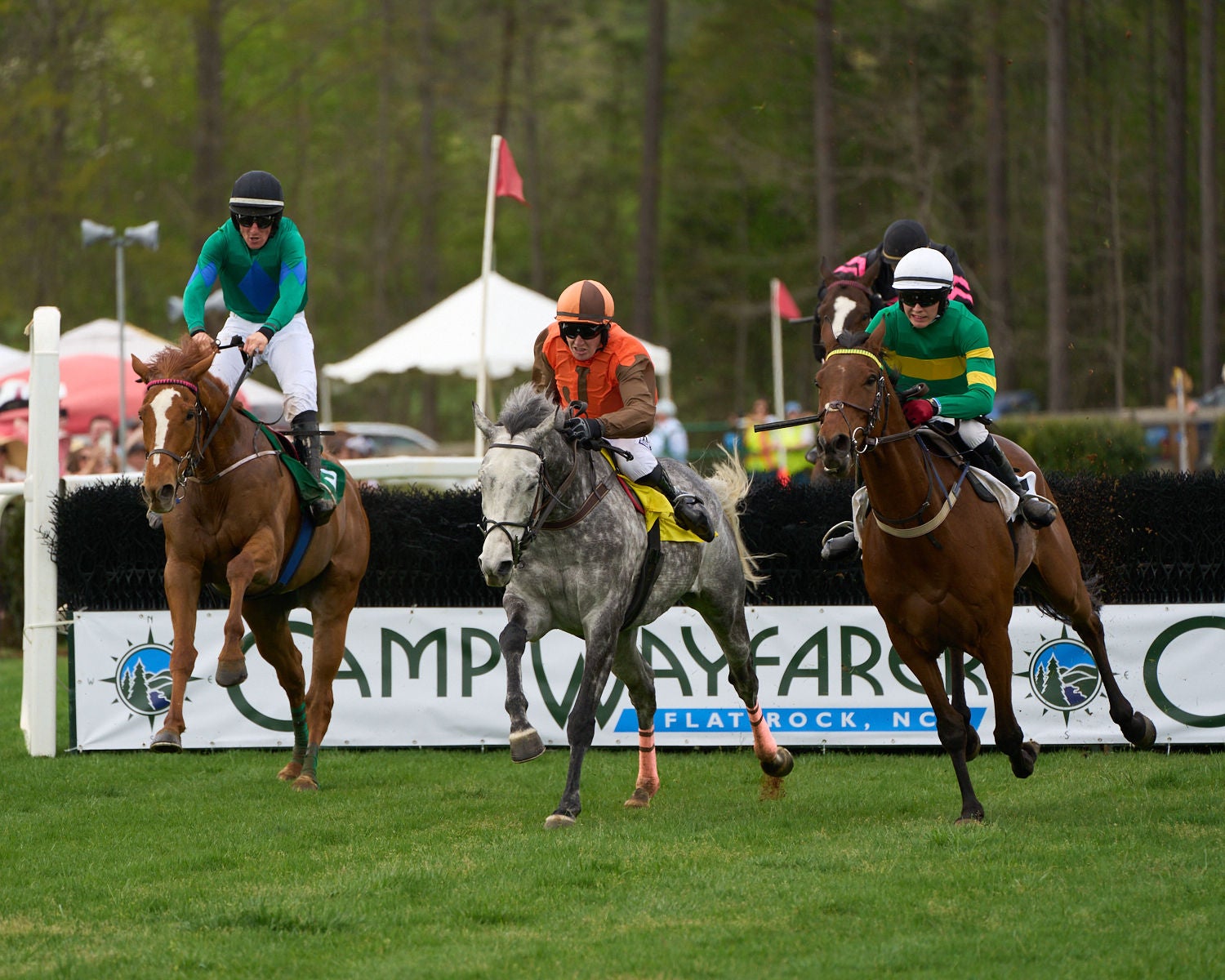The photograph showcases a high-energy horse race set on a lush, green grass field. Three jockeys and their horses dominate the center of the image, with each horse and rider distinctively dressed. On the left, a jockey in green and white rides a brown horse. The central figure is a jockey in white pants and an orange jacket, mounted on a striking gray and white speckled horse. To the right, another brown horse is ridden by a jockey sporting white pants and a green and yellow striped shirt. In the midst of their race, the jockeys appear synchronized, evoking a sense of coordinated competition.

Behind the racing trio, a fourth horse and jockey in a black helmet can be glimpsed, hinting at the extended action of the race. Red flags on poles are interspersed through the background, adding to the competitive atmosphere. Advertisements with banners, including one that reads “Camp Wayfarer,” are visible, indicating potential hurdles the horses need to jump over during the race.

The backdrop features a densely wooded forest, providing a serene contrast to the race's intensity. Larger umbrellas and pavilions suggest an area where spectators might be gathered, offering both shade and a vantage point for viewing the race. The meticulously trimmed grass and the surrounding natural beauty enhance the overall scene, making the photograph a vivid snapshot of an equestrian event set in a picturesque location.